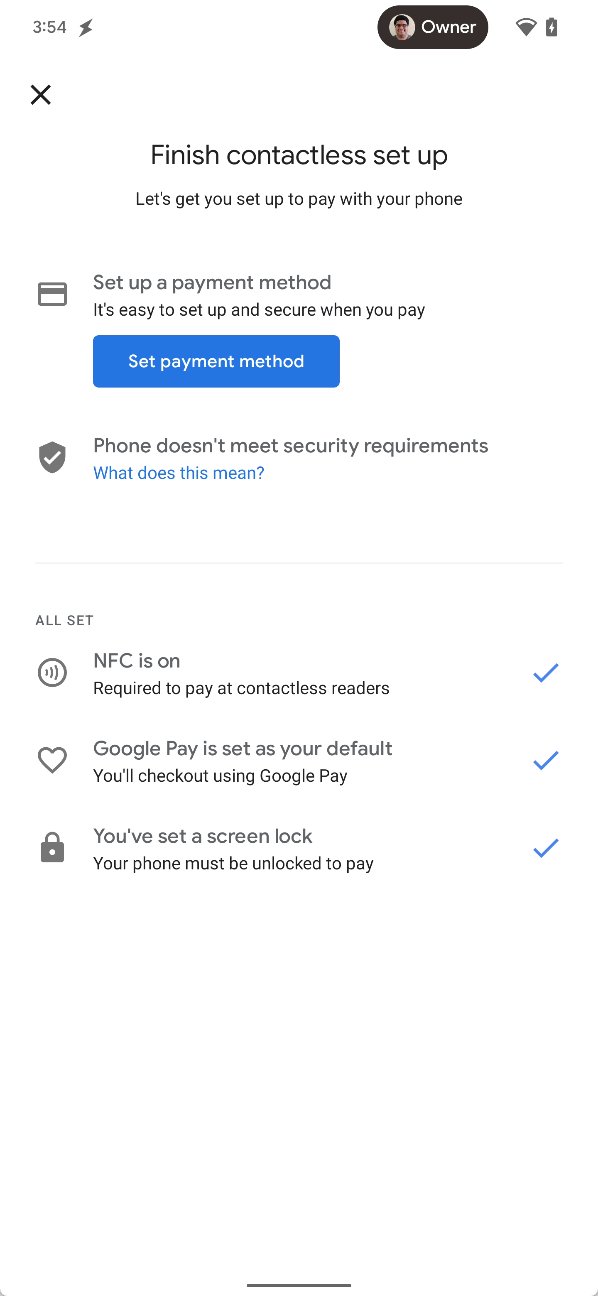The smartphone screen displays a series of notifications and icons at 3:54 PM. The top left corner has a lightning bolt icon indicating a charged battery, and next to it is a small profile image of a man with dark hair who appears to be around 39 years old. To the right of his picture, the word "Owner" is displayed. 

Beneath this, a notification reads "Finished contactless setup" with an invitation to "Set up a payment method." It assures users that it is "easy to set up and secure when you pay," accompanied by a small credit card icon and a blue "Set Payment Method" button featuring a shield and checkmark for security confirmation.

A subsequent message is presented with a warning: "Phone doesn't meet security requirements, what does this mean?" This is followed by confirmation messages:
1. "All set, NFC is on, required to pay at contactless readers" with a blue checkmark.
2. "Google Pay is set as your default. You'll check out using Google Pay," also corroborated by a blue checkmark.
3. "You've set a screen lock, your phone must be unlocked to pay," illustrated with a lock icon.

Additionally, there is a heart symbol, presumably indicating a preference or favorite status. This detailed arrangement of icons and notifications emphasizes Google Pay's activation and readiness features.